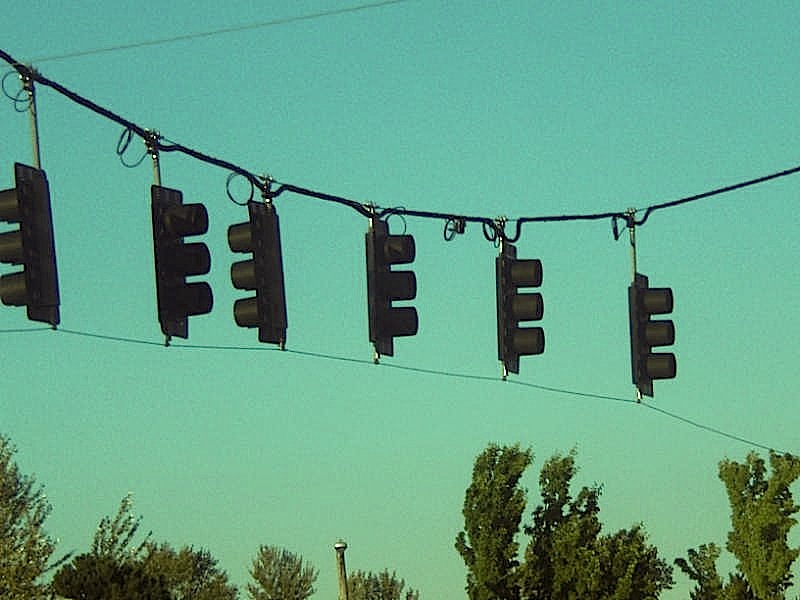The image captures an array of six traditional traffic lights suspended from a black cable that runs across the upper portion of the frame, slightly sagging in the middle. These traffic lights are housed in black casings and each comprises three vertically stacked, unlit signal sections, likely intended for red, yellow, and green lenses. The lights face in various directions: four point to the right, and two to the left, with one light focused in each direction appearing between the two groups. Additionally, a thinner wire can be seen running along the bottom of the traffic lights. The background features a clear, bluish-green sky and the tops of green trees, which appear to be gently bent to the right, suggesting a breeze. The overall arrangement of the traffic lights seems rather haphazard, as none of the lights are illuminated and their varied orientations imply they are not actively directing traffic. No vehicles or street activity are visible below the lights.